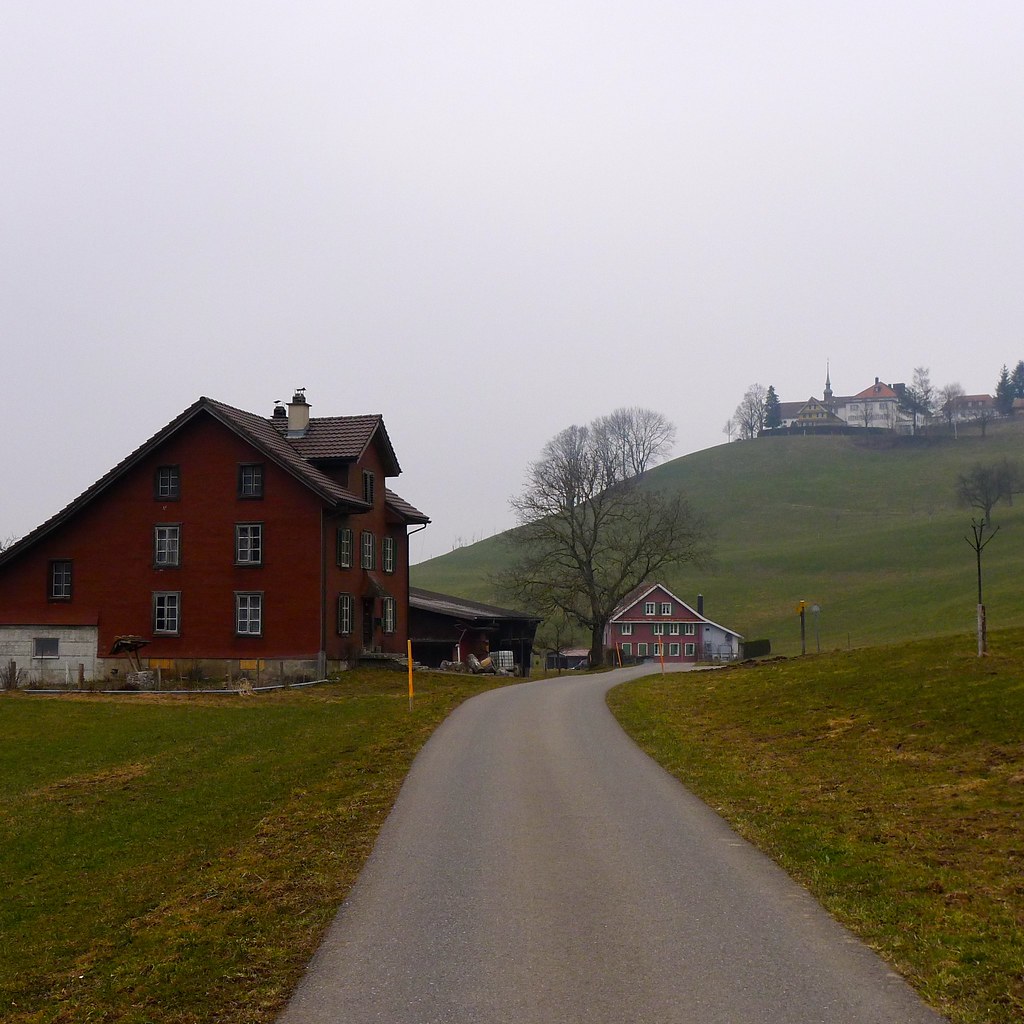The image depicts a rural countryside scene, likely reminiscent of the English countryside. A narrow, winding road ascends a hill, flanked by brownish-green grass. On the left side of the road stands a prominent brick house with a pointed brown roof, featuring three stories of windows arranged in rows. As the road continues upward, another similar brick house with white windows and an attic can be seen. Between these houses, there is a barn-like structure and several leafless trees, indicating a fall or winter season. Further up on the hill, shrouded in fog, another large house is visible. The sky above is a foggy, whitish-gray, adding to the tranquil and somewhat somber atmosphere of the scene.